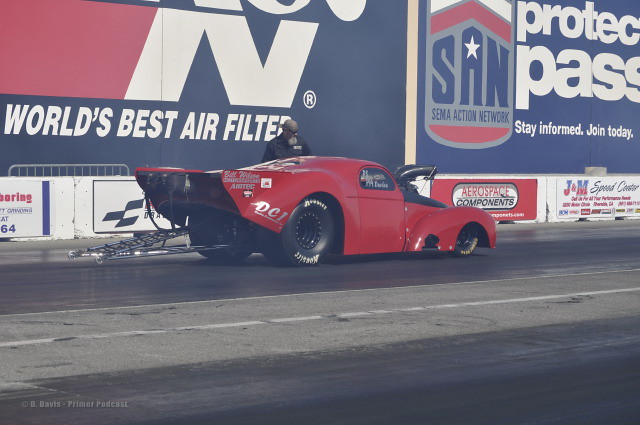The photograph captures a stunning red race car on a racetrack, positioned against a wall lined with various advertisements and billboards. The sleek, polished car, with its low hood, sloping windshield, and dome-shaped roof, extends into a fin-like arrangement at the rear. The vehicle is equipped with large black tires at the back and smaller ones in the front, covered by elaborate curved fenders. The rear prominently displays the phrase "DCI Air Tech." 

In the background, on the wall to the left, there is a dark blue billboard with the phrase "World's Best Air Filter" in large white capital letters, accompanied by a partially visible logo. To the right, a large billboard with a dark blue background displays a banner with a white and red arrow, the acronym "S.A.N." (with a white star in the middle of the 'A'), and the phrase "SEMA Action Network" in blue, followed by "Protect Pass." Below these are a row of smaller rectangular advertisements, including one for aerospace components and another for J&M Speed Center. 

On the black asphalt track, the car appears to be stationary, with a person inspecting its exterior near the left side of the vehicle. The setting sun highlights the pristine finish of the car, standing in contrast against the colorful backdrop of promotional billboards.